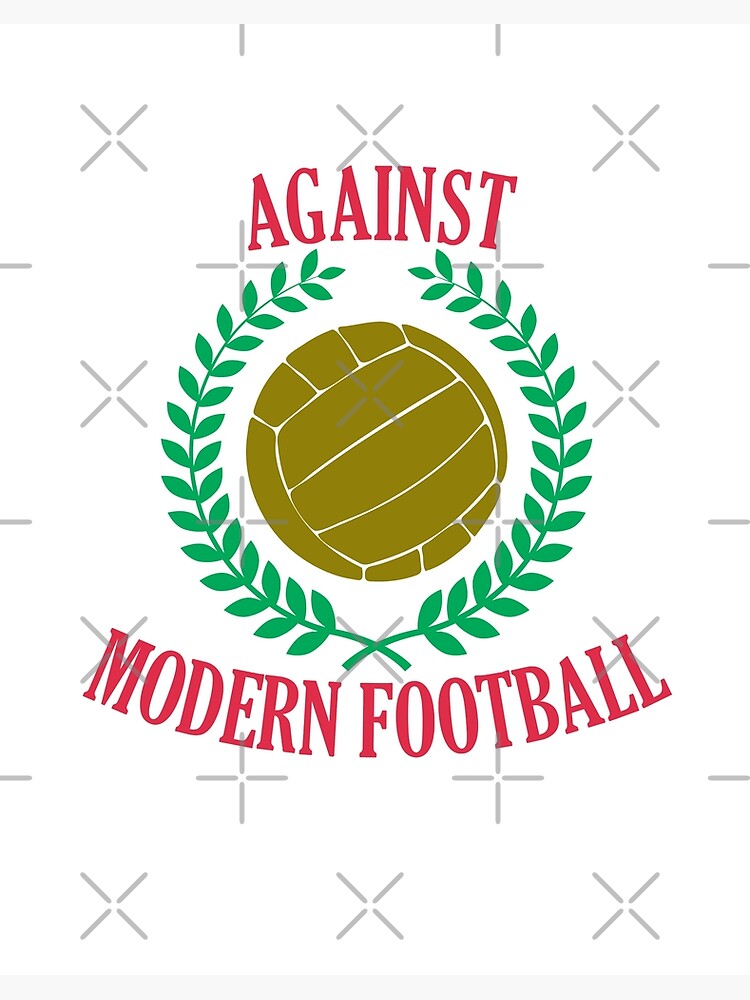This digital poster features a central image of a dark yellow volleyball, surrounded by green compound leaves that nearly enclose the ball, leaving a small gap at the top. The word "AGAINST" is prominently displayed in capital red letters at the top, while "MODERN FOOTBALL" is written in capital red letters at the bottom. The ball, which resembles a soccer ball in its design, has white stripes separating its sections. The poster's white background is adorned with a series of gray X's and plus signs, acting as watermarks distributed evenly throughout the image.